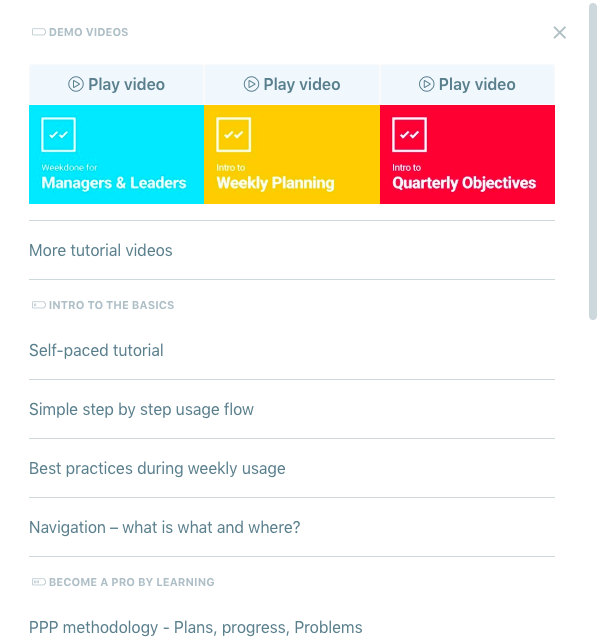The image depicts a tutorial section of an application, presumably a planning or finance app, given its layout. The background is entirely white, creating a clean, minimalist look. In the top-left corner, there is small, very light gray text that reads, "Demo Videos."

Below this header are three video sections, each designed to guide the user through different aspects of the app. Each video section features the label "Play Video" accompanied by a play symbol to its left. The first video section is highlighted with a blue icon and titled "Management and Leaders." The second section, marked with a yellow icon, is labeled "Meeting Weekly Planning." The third section, indicated by a red icon, is called "Quarterly Objectives."

Underneath these video sections is a list of additional tutorial options, organized by horizontal lines separating each item. This list includes:
- "More Tutorial Videos"
- "Intro to the Basics"
- "Self-Paced Tutorial"
- "Step-by-Step Usage Flow"
- "Best Practices During Weekly Usage"
- "Navigation: What is What and Where"

A subsequent section, introduced by another horizontal line, encourages users to elevate their skills by learning the "PPP Methodology - Plans, Progress, Problems." 

Overall, this page serves as a comprehensive guide to help users familiarize themselves with the app's functionalities and best usage practices.